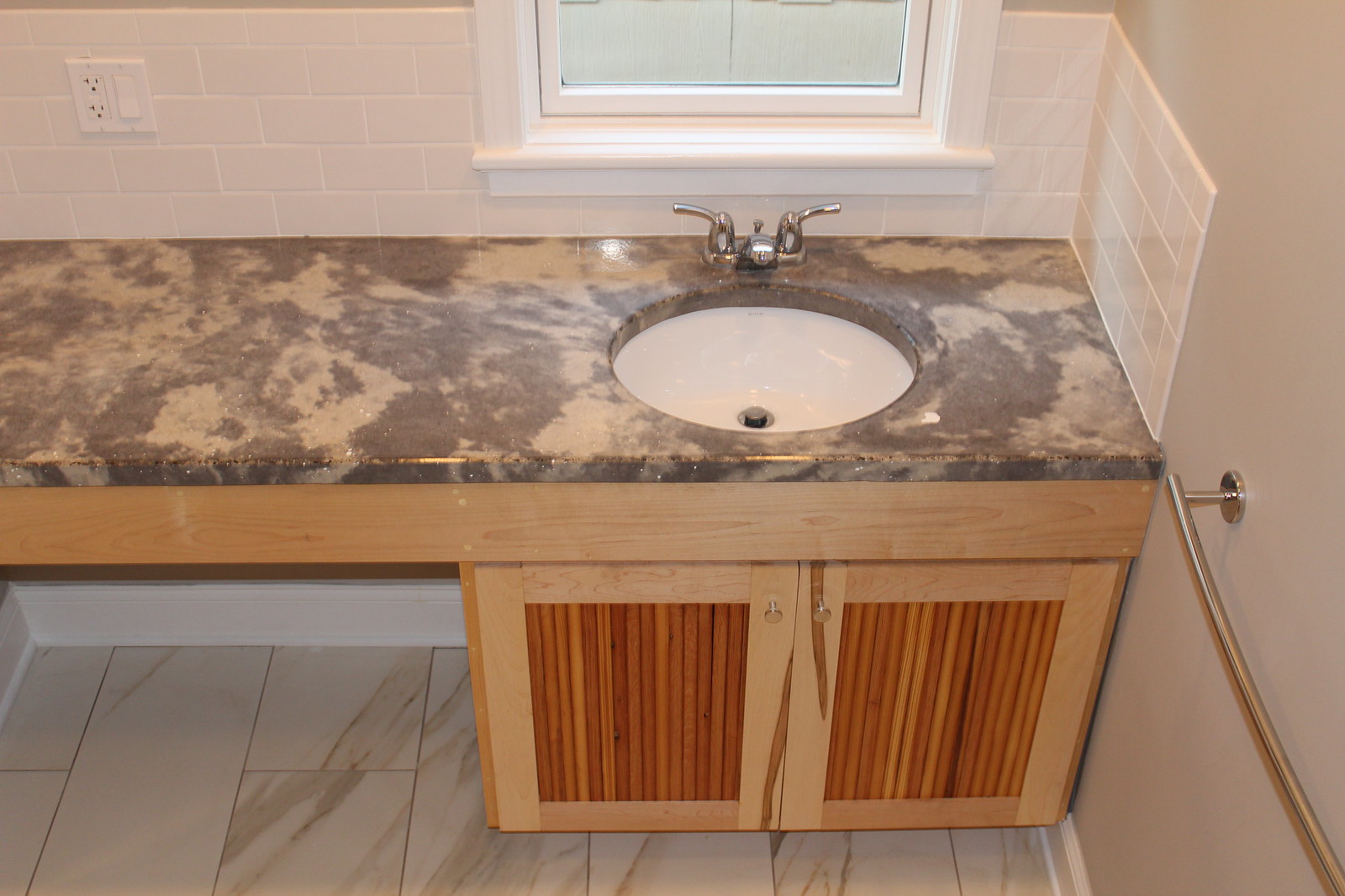Aerial view of a bathroom corner featuring a wash hand basin encased in a cabinet. The basin is a pristine white porcelain fixture, circular in shape, and set into a countertop adorned with a patchwork of brown and very light beige hues. This countertop design adds a touch of rustic charm to the space. The gleaming chrome faucets feature two separate handles, one for hot and one for cold water, accentuating the basin's classic appeal.

Above the sink, the wall is adorned with a mix of white square and rectangular tiles, creating a clean and cohesive look. The floor beneath the sink continues the elegant theme with square and rectangular tiles that resemble white marble, interspersed with intricate gray streaks and specks, giving the floor a luxurious appearance.

The right wall of the bathroom is painted in a warm cream color, adding a soft contrast to the otherwise cool-toned space. Attached to this wall is a towel holder bar, conveniently placed for easy access. 

This carefully curated combination of materials and colors creates a harmonious and inviting bathroom environment.